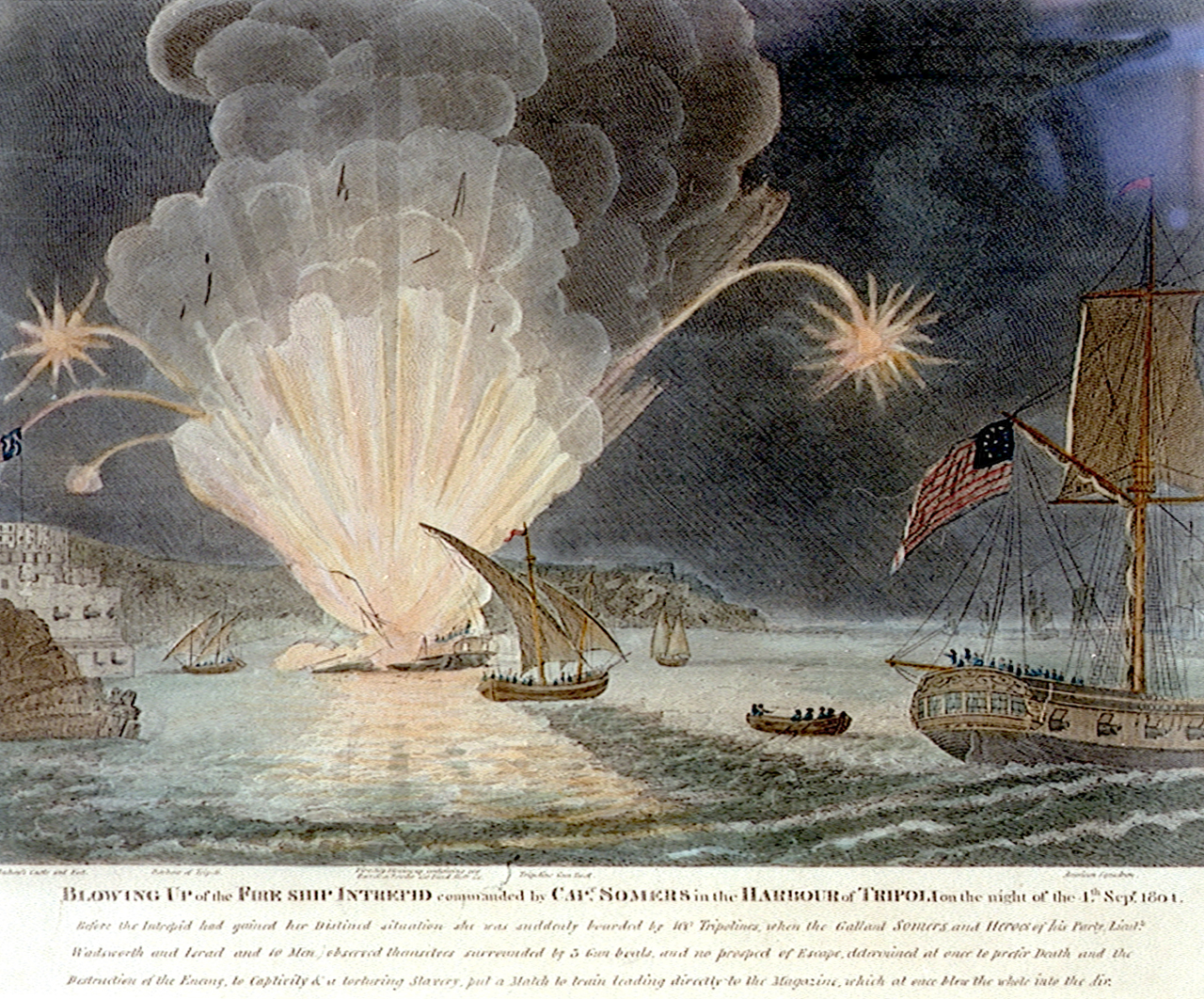The painting captures a famous naval battle during the First Barbary War, specifically the explosion of the fire ship Intrepid, commanded by Captain Richard Somers, in the harbor of Tripoli on the night of September 1st, 1804. The scene is chaotic and dramatic, depicting the American ship with its flag prominently displayed to the right, while the ill-fated Intrepid is centrally positioned and shown exploding, with debris and fragments flying through the air resembling fireworks. The surrounding waters are filled with other vessels, some attempting to flee the destruction, emphasizing the intensity of the battle. Below the painting, a caption provides context, though it's somewhat difficult to read. This detailed and historical artwork might be found in a museum, illustrating an important moment in American naval history.